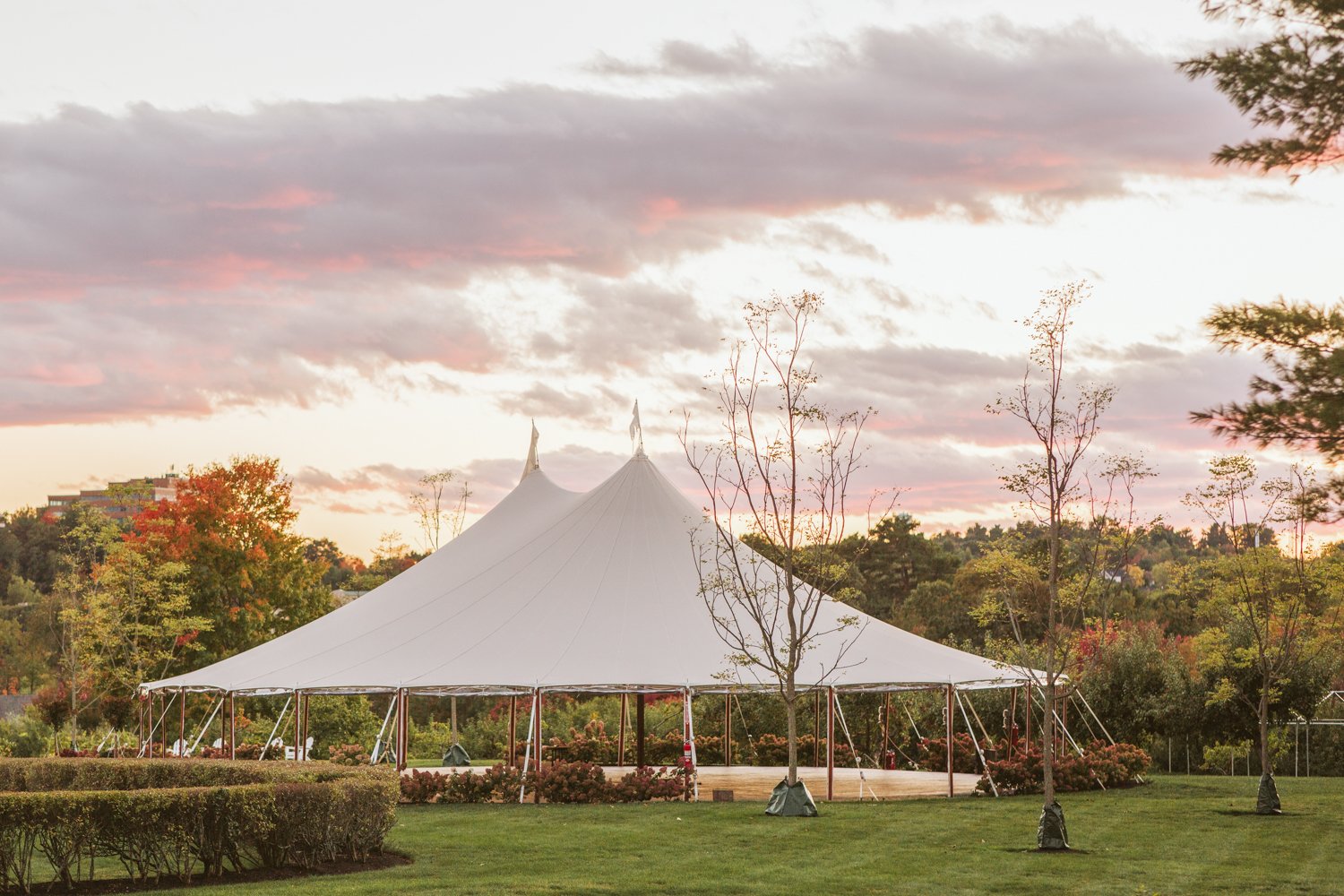This photograph captures a picturesque outdoor setting dominated by a large, white canopy event tent with open sides, positioned in the lower half of the image. The tent has two peaks, each adorned with small white flags, and is supported by brown-colored beams around the exterior. The ground under the tent appears to be a sand-colored paved area, situated in the middle of a neatly mowed lawn or park setting. The sky above is filled with fluffy clouds tinged with pink and orange hues, suggesting the warm light of either a sunrise or sunset. The beautifully manicured lawn features mow lines and is accentuated by various shrubs, particularly in the lower left corner, and a few smaller trees on the right. The background transitions to denser tree cover, with trees showing the vibrant fall colors of reds, oranges, yellows, and greens. The overall atmosphere suggests preparation for a special event, possibly a wedding or banquet, emphasizing its organized and well-maintained appearance.